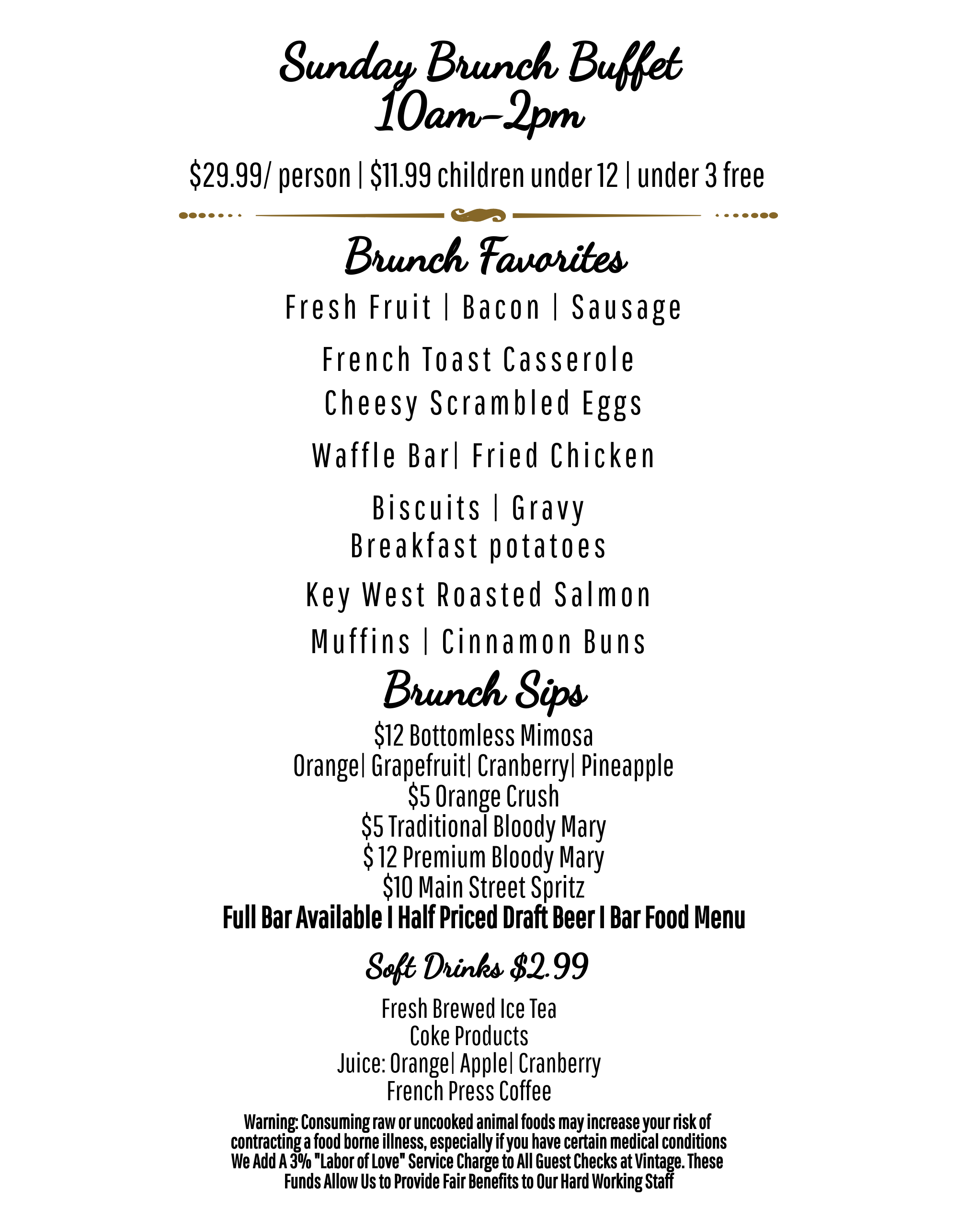This image features a detailed menu for a Sunday brunch buffet, set against a pristine white background with black font. The buffet runs from 10 a.m. to 2 p.m., priced at $29.99 per person, $11.99 for children under 12, and free for kids under 3. The "Brunch Favorites" section includes a variety of delectable options, such as fresh fruit, bacon, sausage, French toast casserole, cheesy scrambled eggs, a waffle bar, fried chicken, biscuits with gravy, breakfast potatoes, Key West roasted salmon, muffins, and cinnamon buns. 

The "Brunch Sips" section offers a selection of beverages: $12 bottomless mimosas available in orange, grapefruit, cranberry, and pineapple flavors, $5 orange crush, $5 traditional Bloody Mary, $12 premium Bloody Mary, and $10 Main Street Spritz. Additionally, there's a full bar available, half-price draft beer, a bar food menu, $2.99 soft drinks, fresh brewed iced tea, Coke products, and various juices including orange, apple, and cranberry, as well as French press coffee.

A small print note at the bottom of the menu warns that consuming raw or undercooked animal foods may increase the risk of foodborne illness, especially for individuals with certain medical conditions. Moreover, a 3% "Labor of Love" service charge is added to all checks at Vintage to provide fair benefits for the hardworking staff.